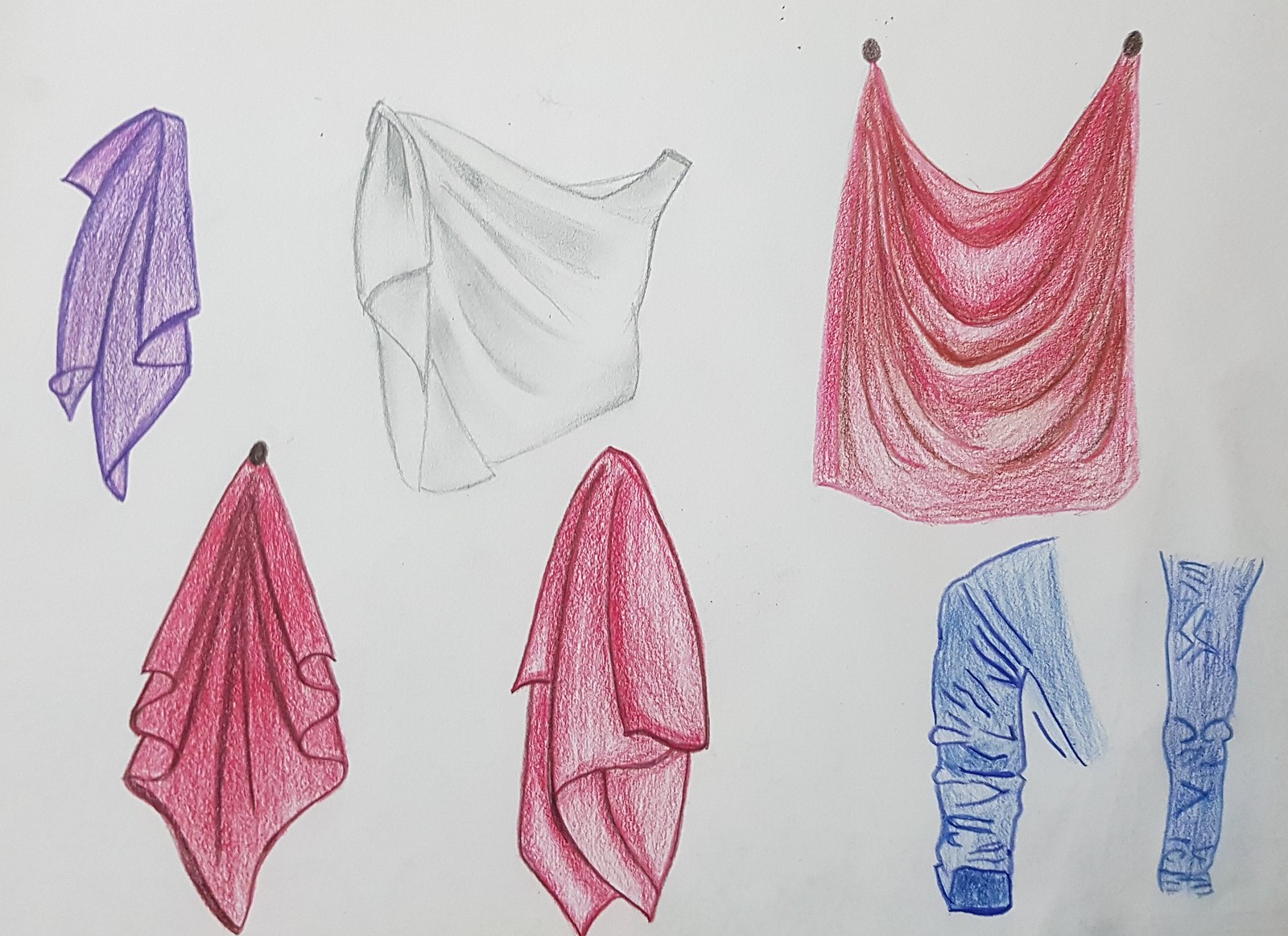A hand-drawn illustration, seemingly created using crayon or pencil, showcasing an array of objects distinguished by their varied shapes and colors. In the upper left corner, a draped purple scarf, approximately two to three feet in length, cascades delicately. Adjacent to this, a sizable white object which could either be a tank top or possibly a bedding item adds an air of mystery. Further along, a red object spreads out in a flowing manner, likely depicting a blanket. Completing the ensemble, another item, also resembling a blanket, elegantly descends into a V formation. This compilation of sketches captures a diverse collection of fabrics and textures, inviting viewers to imagine the tactile sensations each item might evoke.